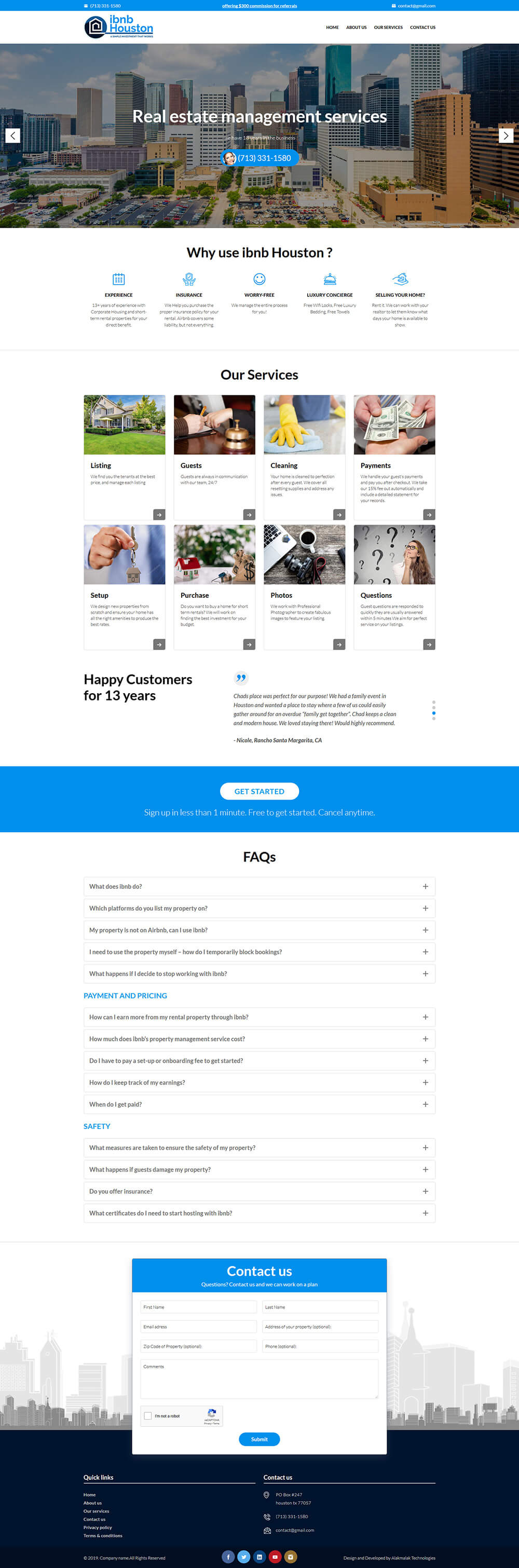The image is a screenshot from a website called "I B&B Houston," which specializes in real estate management services. The background of the image showcases part of the Houston city skyline, featuring numerous tall buildings and a parking lot filled with cars under a beautiful sky. The website's navigation bar includes drop-down menus with options such as Home, About Us, Our Services, and Contact Us. 

At the top of the page, there's a noticeable blue bar prominently displaying the company’s phone number alongside an image of a customer service representative wearing a headset. Below this, the website highlights reasons to choose I B&B Houston, emphasizing their experience, insurance options, worry-free luxury, and conscientious home selling.

Further sections on the webpage feature client testimonials celebrating 13 years of happy customers, a Frequently Asked Questions (FAQ) area, and a Contact section. The bottom part of the website includes quick link options for easy navigation.